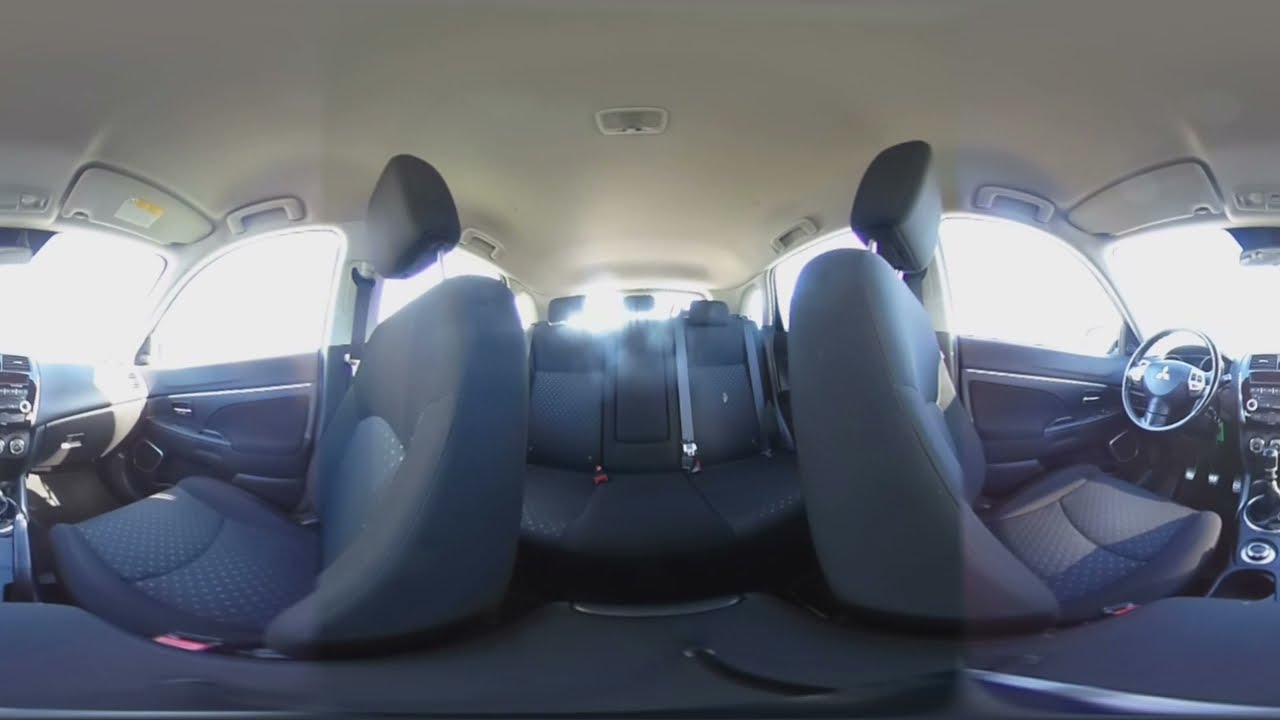The image is a panoramic, 360-degree interior shot of a Mitsubishi vehicle. Centered in the photograph is the back row, with three gray fabric seats. Uniquely distorted by the 360-degree view, the driver's seat on the right appears to be oriented completely to the right, showcasing the steering wheel and driver controls such as the stick shift. Similarly, the front passenger seat on the left seems to be turned completely to the left. A ray of light illuminates parts of the interior, causing a gradient from darker to lighter gray on the front seats. The roof of the vehicle is a light tan color. The car is completely empty, and out the windows, the daylight renders the exterior pure white. The image is rectangular, with dimensions of approximately six inches wide and four inches tall, bordered by a thin black header and footer that collectively occupy about half an inch of the overall image height.